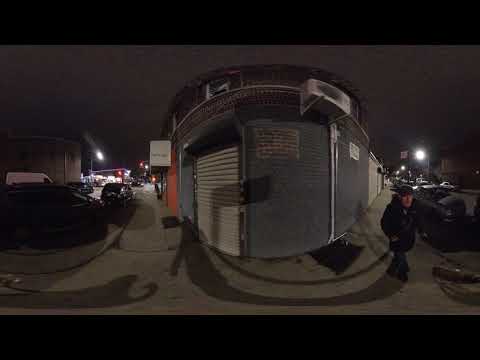The photograph captures a nighttime street scene through a distorting lens, creating a convex effect that warps the central part of the image. The central portion is flanked by black frames on the top and bottom, encompassing about three-quarters to four-fifths of the overall view. The street scene features a series of buildings and storage units that curve unnaturally due to the lens distortion. A prominent blue building with gray corrugated metal roll-up doors and an air conditioner unit protruding from the top dominates the center of the image. Streetlamps illuminate the scene faintly, casting light on parked cars and illuminating the sidewalk, which curves around a street corner. 

In the foreground on the right side of the image, an older gentleman wearing a black helmet, dark jacket, pants, and shoes is walking towards the camera, his shadow following the curvature of the building behind him. The sky suggests it is either night or approaching night, painted in dark charcoal gray rather than pitch black. Red and white lights adorn the sides of the buildings, adding splashes of color to the otherwise dimly lit street. Farther down the street, additional cars and streetlamps can be seen, contributing to the urban atmosphere of the scene.